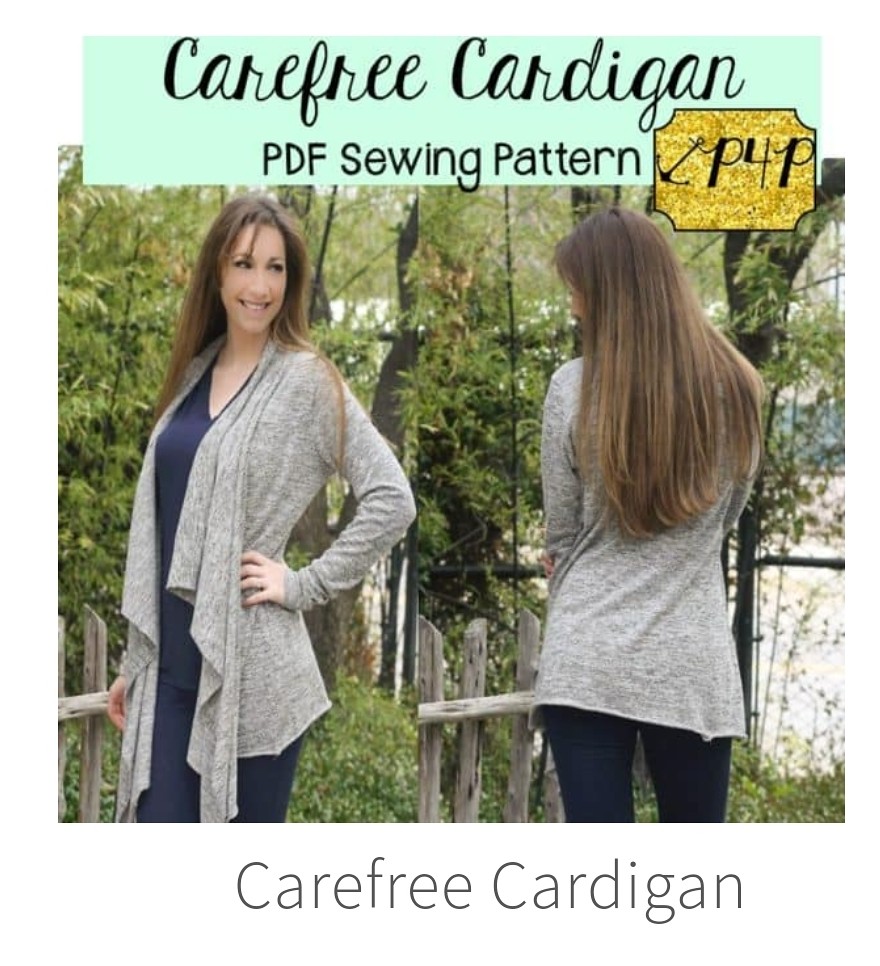This advertisement showcases a detailed visual of a gray cardigan in a serene outdoor setting. The main image is divided into two halves. On the left, a woman with long brown hair is seen facing the camera. She is wearing a long gray cardigan over a navy blue top and matching pants, with her left hand posed on her hip and her right hand by her side. She stands in front of a small, rickety wooden fence, framed by a background filled with trees that allows some light to filter through.

On the right half of the image, another view captures the back of the same woman, showcasing her long hair cascading down to the middle of her back, highlighting the design of the cardigan from behind. This perspective confirms that both views are of the same person.

At the top of the image, a teal banner with cursive black text reads, "Carefree Cardigan" followed by "PDF Sewing Pattern" in print below. In the upper right corner, a small red square featuring a black anchor symbol is labeled with "P4P". The bottom of the image reiterates "Carefree Cardigan" in a blue sans-serif font.

The calm and inviting scenery, coupled with the clear and detailed presentation of the cardigan, effectively emphasizes the design and comfort of the garment, making it an appealing ad for potential customers.